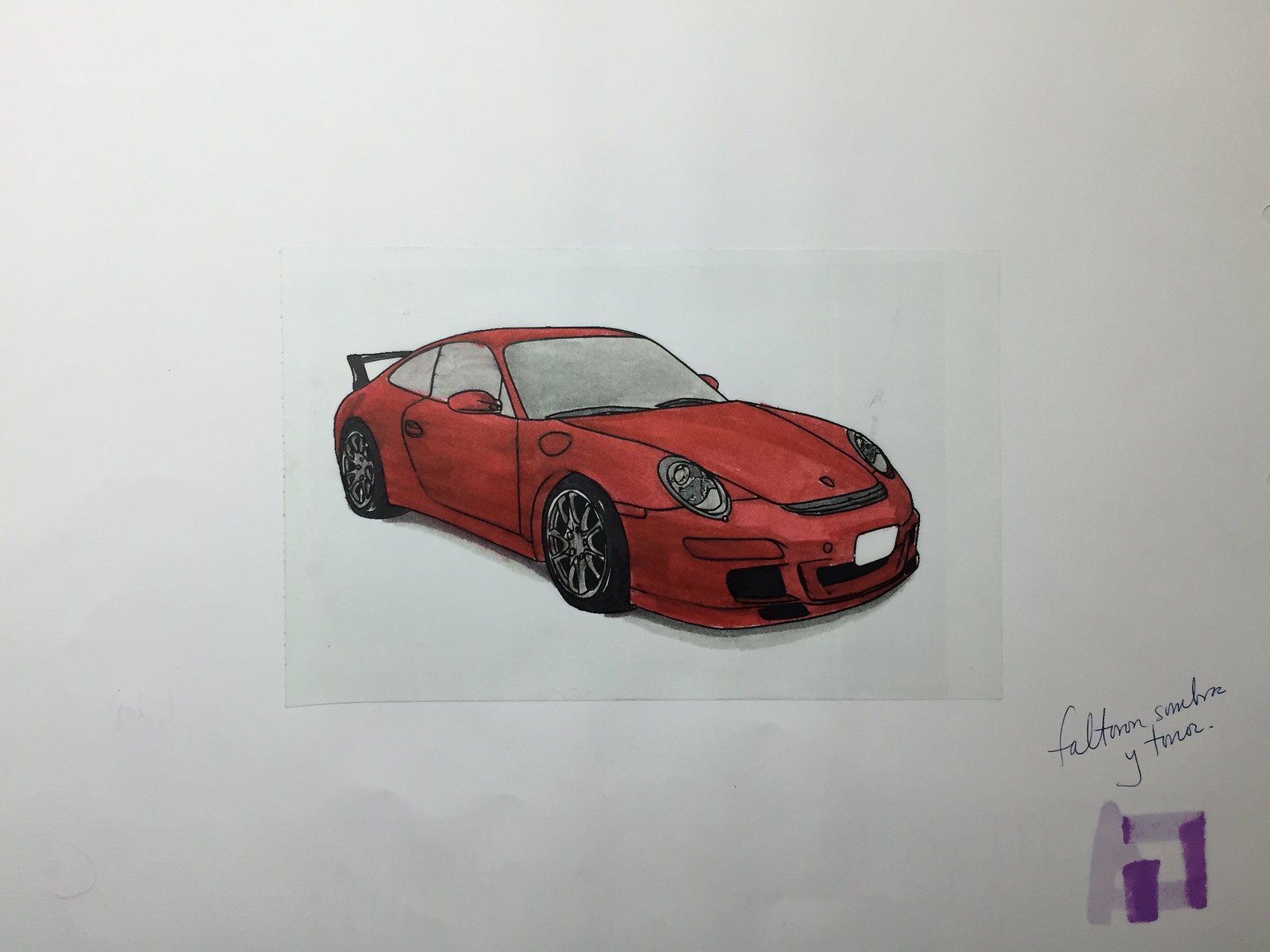A detailed sketch of a sleek, red Porsche sports car dominates this large piece of paper. The car features a low-slung coupe design with two doors, embodying the essence of a high-performance vehicle. A white license plate adorns the front, adding to its realistic depiction. Although the overall paper is white, the paper seems to have a slightly grayish tint, contrasting with the bright red of the car.

The car is positioned at a northwest-to-southeast angle, making it appear as if it’s parked and angled towards the viewer. The windows are rendered in a metallic gray, giving them an opaque look and forgoing any interior details. A stylish spoiler sits at the rear, enhancing the car's sporty aesthetic.

In one corner of the sketch, there’s a handwritten note in an unidentified language, followed by what seems to be initials – possibly "AP" – written in light lavender with some darker streaks incorporated. The car, meticulously drawn with minimal details, stands out as a stationary figure, exuding a snazzy, sophisticated vibe true to Porsche’s reputation.